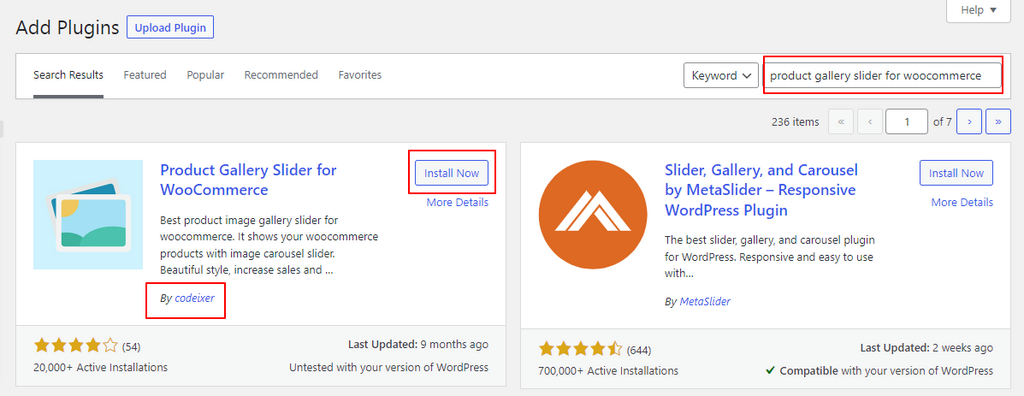The image depicts a web interface for adding plugins, specifically for WooCommerce. 

On the left-hand side, there's a black rectangular background with the text "Add Plugins" in white. Below this, within a blue-bordered box, the option "Upload Plugin" is presented in blue.

On the right-hand side, a gray "Help" button is visible. Below it, a white rectangular search bar contains the black, underlined text "Search results." Underneath this, there are categories labeled "Feature," "Popular," "Recommended," and "Favorite."

Further down, a keyword text box is shown, followed by another text box outlined in red without a clear label. 

The main content includes a section titled "Product Gallery Slider for WooCommerce." The right side of this section is marked "236 items" in black. Adjacent to this, there is a box labeled "1 of 7."

Within the plugin listing, a blue-bordered button labeled "Product Gallery Slider for WooCommerce" is present on the left, accompanied by a blue "Install Now" button within a gray rectangular outline. Both these elements are surrounded by another red box. Below this, a link "More Details" in blue is available, and at the bottom, there's a "Buy" button next to the blue text "CODEIXER," also encased in a red box. This listing indicates "20,000 Active Installations" in black at the bottom.

Adjacent to the main section, another plugin titled "Slider Gallery and Carousel by MetaSlider" is presented. It features a blue "Install Now" button, a "More Details" link, and a "Buy MetaSlider" option, all in blue.

Overall, the interface is focused on listing and providing details for various WooCommerce gallery slider plugins, with some elements highlighted by red boxes for emphasis.